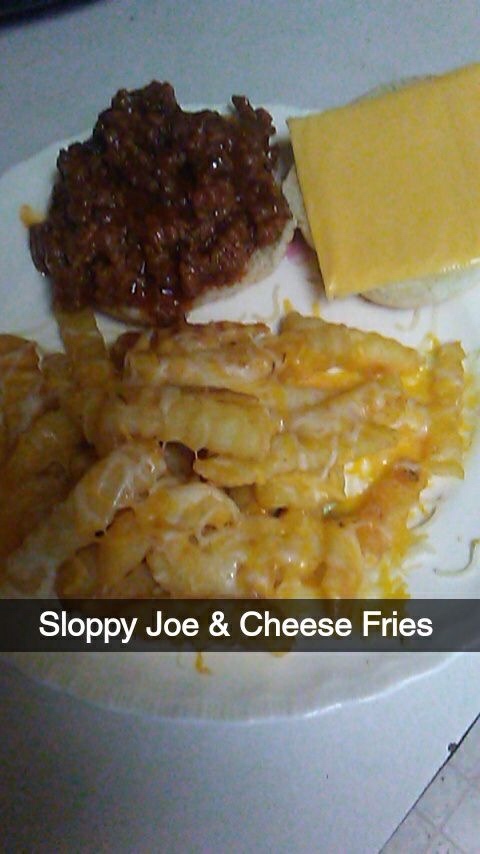The photo depicts a white round plate positioned on a white surface, likely a table or countertop, covered with a white tablecloth or napkin. On the plate, there are two white hamburger buns: the bun on the left is topped with a sloppy joe mixture, consisting of ground beef in a brownish-red sauce, while the bun on the right holds a slice of unmelted American cheese. Below the buns, the plate is filled with crinkle-cut fries smothered in melted cheese that appears to be a blend of both cheddar and mozzarella, exhibiting orange and white hues. Spanning horizontally across the bottom of the plate is a slightly transparent black banner with slim, white text that reads "Sloppy Joe and Cheese Fries." The image has a grainy quality, suggesting it might be an older photograph. The background features a white table edge in the upper left corner and a dark brown void behind it, with white tiles visible in the lower right corner.